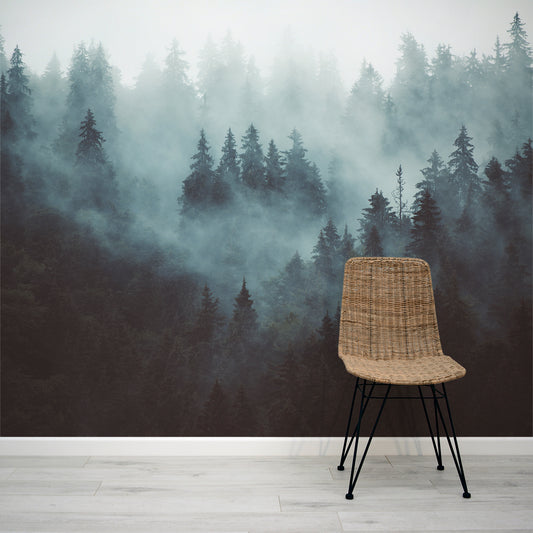The image captures a serene living room scene early in the morning, featuring a captivating forest mural dominating the wall. The mural, likely a photograph, depicts an expansive view of dark green, evergreen trees shrouded in a thick layer of white fog, evoking the misty ambiance of the Appalachian or Smoky Mountains. The sky above the treetops remains a muted gray, enhancing the ethereal atmosphere. In front of this striking backdrop, a wicker chair with angled black metal legs sits upright, positioned slightly to the right of the center. The chair is a light brown or beige color and contrasts with the pristine white panel flooring and white wall trim beneath the mural. The photograph seems to be a deliberate composition to highlight the dramatic interplay between the natural landscape depicted in the mural and the modern simplicity of the chair and floor, creating an intriguing and peaceful focal point within the room.